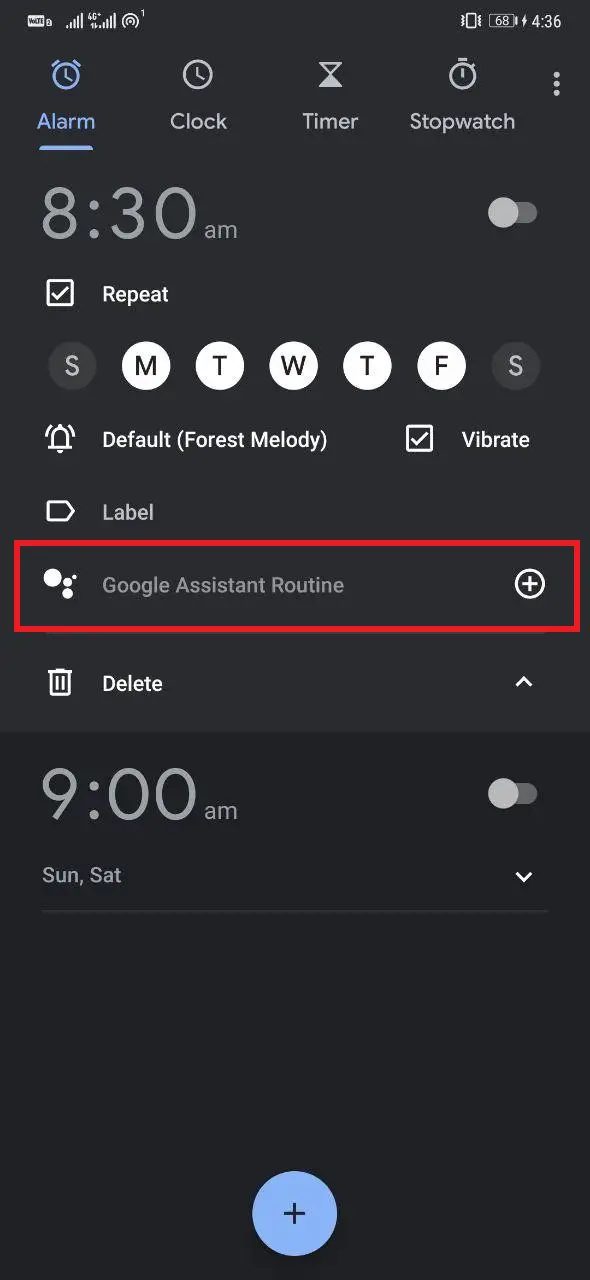This image captures the alarm and clock interface on a smartphone set to dark mode. The screen displays full service, full battery, full Wi-Fi, with a hotspot active, and the phone is on vibrate. The time is 4:36, and screen recording is active. The battery level is at approximately 60%. The dark mode interface features a black background with gray text. The app's options include Alarm, Clock, Timer, and Stopwatch, with the Alarm tab selected.

At the top, an alarm is set for 8:30 AM, but it is currently turned off. The alarm is scheduled to repeat on weekdays (Monday through Friday), indicated by highlighted circles for these days. The alarm is set to play the default "Forest Melody" sound, and the vibrate option is enabled. Below the alarm settings, there's an option to add a label for the alarm, currently labeled "Google Assistant Routine" with a red box and a plus sign next to it. There's also a trash can icon labeled "Delete."

Another alarm is set for 9:00 AM on weekends (Saturday and Sunday), but it is not expanded or turned on. At the bottom of the interface, there's a plus sign to add additional alarms.